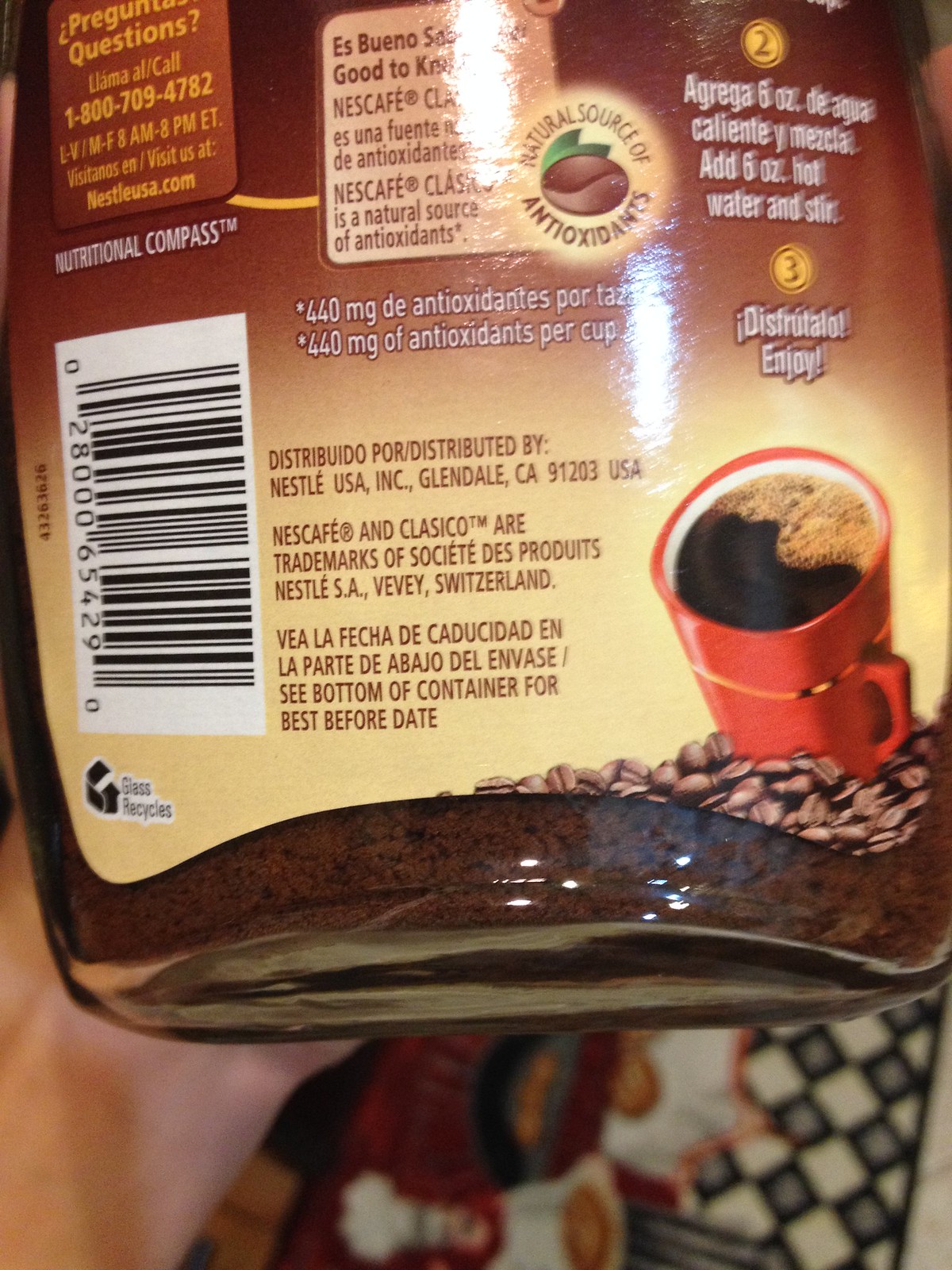A close-up image features a foodstuff jar, likely a coffee jar, held from the bottom left corner by a hand with medium-light skin. The background is blurred, showcasing various textures and colors, including blue and white diamond patterns and a brown area in the middle. The jar itself displays different shades of brown, with a white barcode on the left side. The text on the jar appears in yellow and brown hues. On the bottom right, there's an image of a coffee cup, half in shadow, filled with coffee and surrounded by coffee beans. Prominently displayed in white text on the jar, it reads "400 mg of antioxidants per cup." Additional text indicates that the product is distributed by Nestle, providing various company details. An upper right corner text in white offers a brief usage instruction: "Add six ounces of hot water, stir, and enjoy."